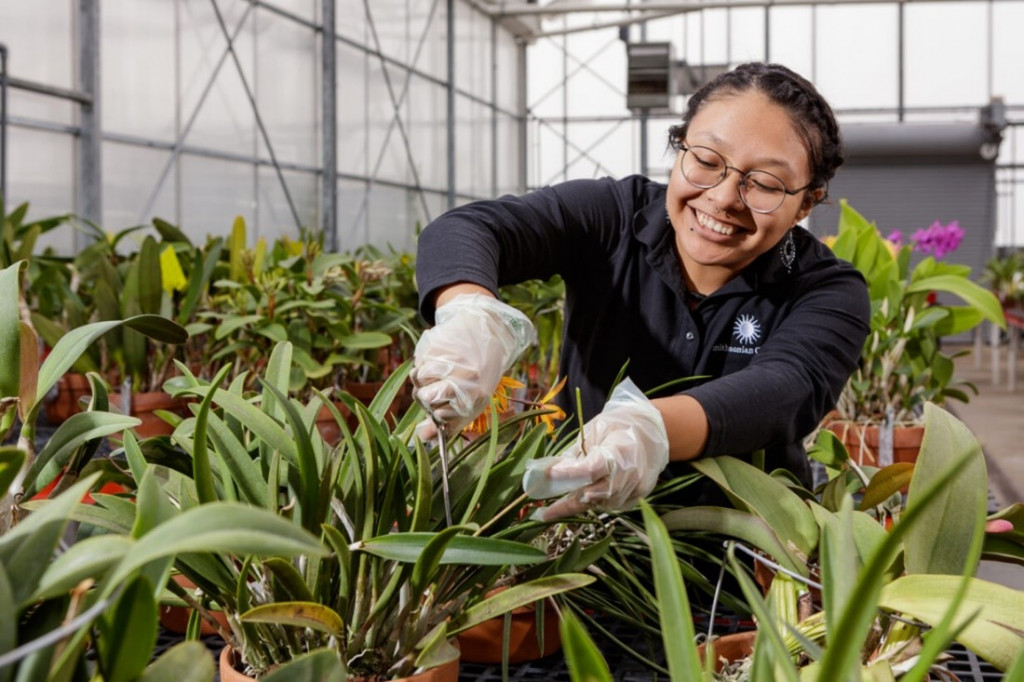The image captures the vibrant scene of a smiling Hispanic woman with dark, tied-back hair, wearing round dark-framed glasses, and dressed in a navy blue, long-sleeve shirt with a collar and an illegible insignia resembling a sun on the upper right side. She is in a bustling greenhouse, surrounded by an abundance of plants in terracotta pots. Her outstretched hands, covered in clear plastic gloves, are engaged in trimming or arranging the foliage in front of her. To her left, the floor is partially visible and appears glossy, possibly linoleum, while the background features transparent walls supported by silver metal framing. The backdrop of the greenhouse showcases a variety of plants, including a prominent cluster of yellowish-orange flowers right in front of her and a notable purple flower visible on her right. Her joyful expression and the meticulous attention she gives to the plants emphasize her enjoyment and dedication to her work.